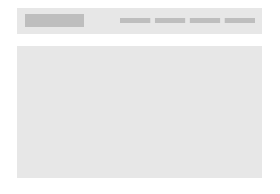The image depicts a solid gray background with a small, narrow rectangular strip of a slightly darker gray shade. Within this strip, there is a smaller, darker gray rectangle positioned centrally. Additionally, there are four even smaller dark gray rectangles aligned vertically, neatly spaced and creating a structured pattern.